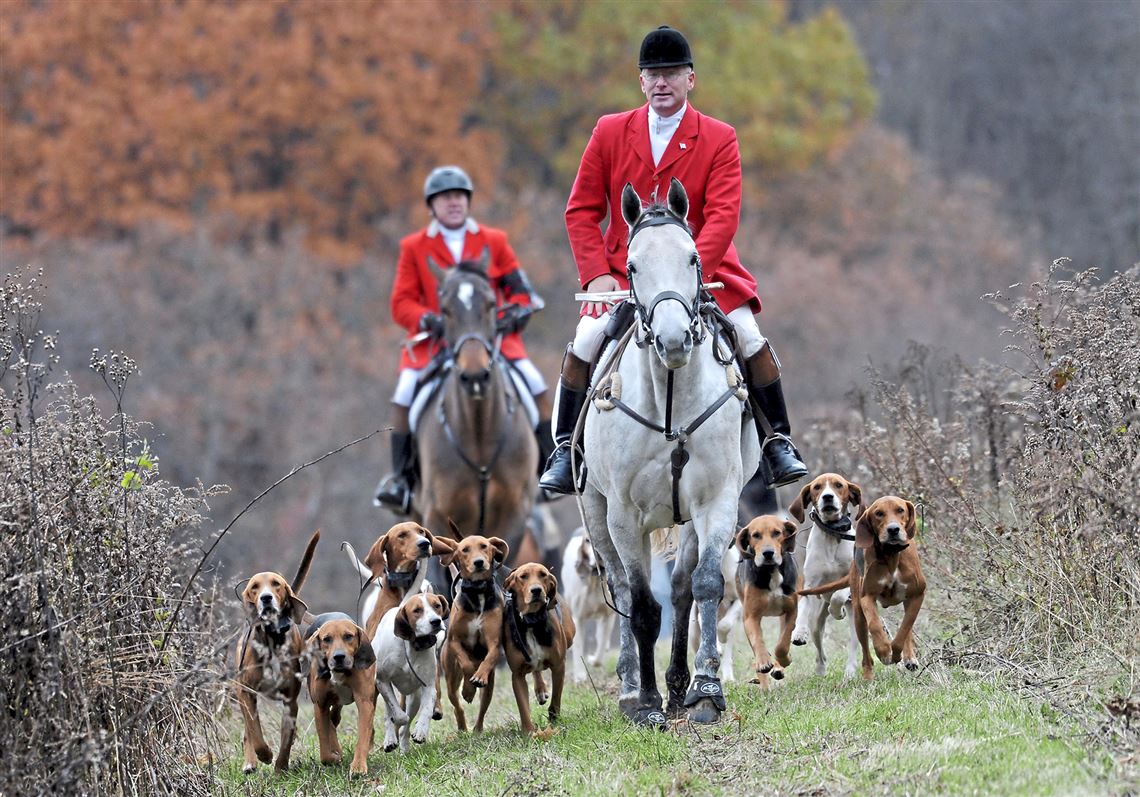The photograph depicts two men on horseback, leading a hunting party along a grassy path bordered by greyish, dead bushes and autumn foliage in varying shades of green and orange. In front, a man riding a white-grey horse is dressed in traditional riding gear: a black riding cap, a bright red coat, white pants, and black leather boots. To his left and slightly behind, another man, identically outfitted but sporting a black helmet instead of a hat, rides a brown horse with a white spot on its head. Surrounding their horses, a dozen black, white, and brown hound dogs trot along, possibly beagles or dachshunds, each with black collars. In the background, vibrant fall trees rise up against a hill, creating a picturesque autumnal setting. The bright red riding coats of the men stand out vividly against the natural scenery, indicating a mid to late autumn hunting excursion.